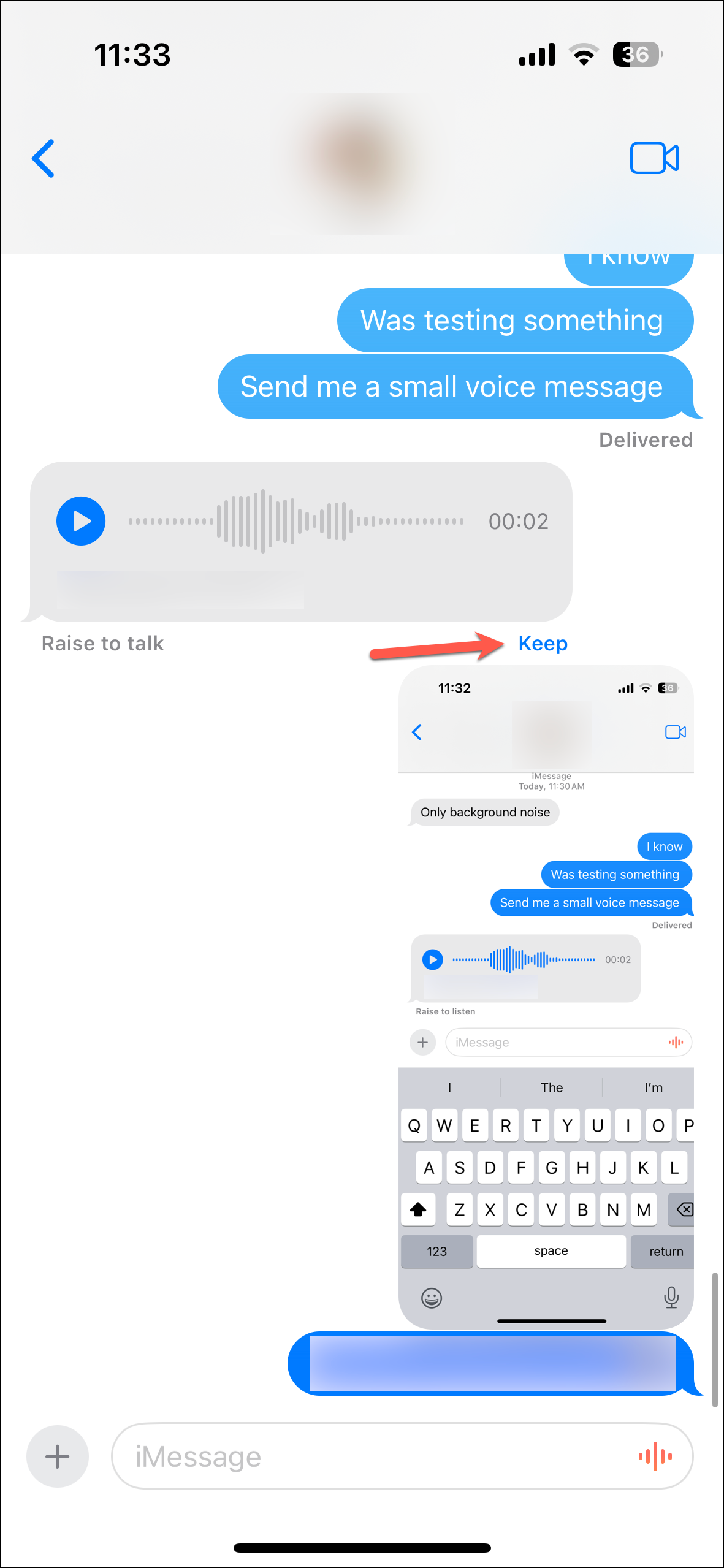In this image, we observe a detailed screenshot of a text message exchange displayed on a cell phone screen. The top section of the image shows the phone's status bar, including the time, Wi-Fi signal strength, and battery level. Below the status bar is a conversation with messages in blue text bubbles. The messages read, "I know" followed by "was testing something" and "Send me a small voice message" spread across three separate bubbles. Featured prominently in the exchange is a blue play button indicating a voice message, with a label beneath it that says "raise to talk" suggesting an interactive function. A red arrow points to blue text that reads "keep," possibly highlighting an option to save the voice message. Additionally, the same screen is captured again within the image as a screenshot, complete with a visible text exchange, implying that the screenshot was either accidentally or deliberately taken and shared within the conversation.